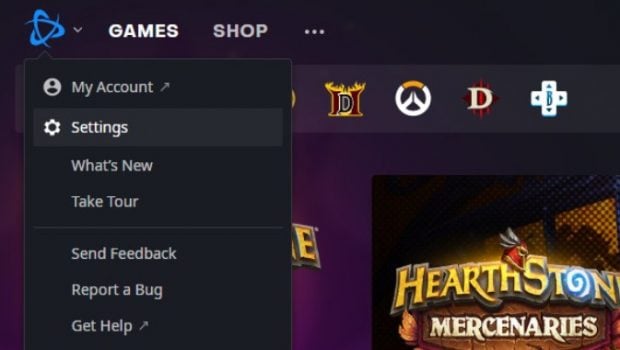This is a detailed screenshot of an unspecified web page with the title "Games and Shop" at the top. The page features a vertical menu on the left side with options labeled "My Account," "Settings" (currently selected), "What's New," "Take Tour," "Send Feedback," "Report a Bug," and "Get Help." To the right of the menu, there are several distinct icons arranged in a row:

1. An icon featuring two flaming pillars flanking a black uppercase 'D.'
2. A white circle with an orange top section and two diagonal areas that converge in the center.
3. An uppercase 'D' with three vertical red lines behind it.
4. A white video game D-pad with a 'B' in the center.

At the very bottom of the image, partially cut off, there is a section labeled "Hearthstone Mercenaries," with the 'O' in 'stone' depicted as a glowing blue spiral. The screenshot does not include any people, animals, buildings, plants, flowers, or trees. The dimensions of the image are wider than it is tall.